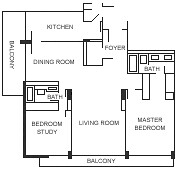This line drawing floor plan depicts a two-bedroom, two-bathroom dwelling. At the front of the image, there is a balcony that provides outdoor space. Directly behind the balcony, to the left, is a versatile room that can function as either a bedroom or a study. This room has access to a shared bathroom that is also accessible from the hallway. 

In the center of the drawing lies the living room, serving as the main communal area of the home. On the right side, the master bedroom features an ensuite bathroom, providing privacy and convenience, as this bathroom is not shared with other parts of the dwelling.

Moving further back, behind the multifunctional bedroom/study, is the dining room, which facilitates meal times and gatherings. Directly behind the dining room is the kitchen, efficiently placed for easy access from the dining area. Flanking this central living space, there is another balcony on the left side, adding additional outdoor space, and a foyer to the right, offering a welcoming entrance to the home.